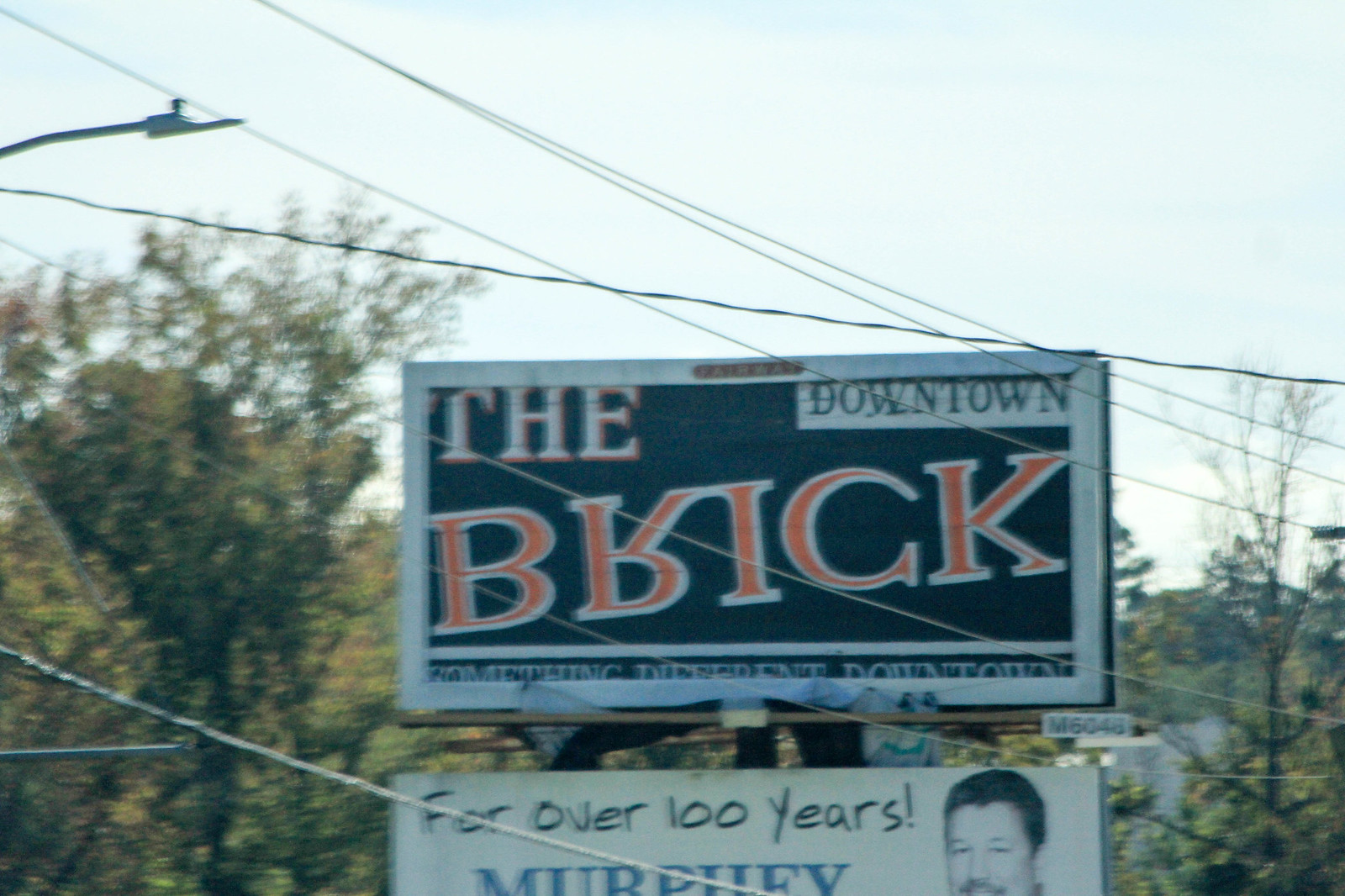In this somewhat blurry photograph taken on an overcast afternoon, two advertisement billboards are prominently displayed against a gray, cloudy sky. The scene is crisscrossed by electrical wires, and the background features trees that appear to be transitioning into fall, with leaves of varying colors. The top billboard has a dark gray or black background with white and red lettering. It reads "the brick" with a quirky upside-down "R." In the upper right corner of this billboard, a small box features the word "downtown" in black letters on a white background. Below "the brick" text, a line states "something different downtown." The second billboard beneath it is entirely white, showcasing an image of a smiling man with dark hair and a mustache. This lower sign reads "for over 100 years!" with "Murphy" highlighted in blue.